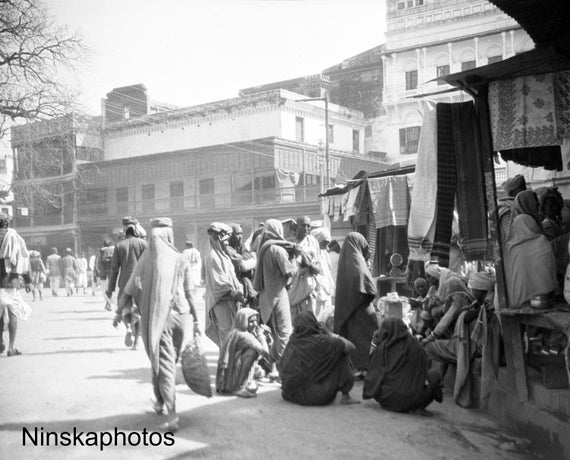This black-and-white photo, credited to Ninska Photos according to the bottom left corner caption, offers a rich and detailed glimpse of a bustling Middle Eastern marketplace. The scene is somewhat faded, giving it a vintage, historical feel. The marketplace is set in front of a backdrop of low-rise buildings that vary in shades of white and dark-colored stone, ascending in height from left to right. Among them, there is a striking three-story building with a dark facade interspersed with white.

The street, likely made of dirt, is teeming with life. Approximately 100 individuals are captured in various activities; some are seated on the ground while others walk or stand in groups. Men dressed in turbans and shawls and women draped in large blankets or capes wrapped around their heads and shoulders are part of the vibrant crowd. A focal point is a vendor booth on the right-hand side, attracting attention with tapestries hanging on boards. Some of these tapestries are displayed higher up, perhaps atop a small stage or structure.

A small metal roof offers partial cover to part of the marketplace, hinting at a central or busy area. Electric lines run prominently through the scene, and a leafless tree on the left-hand side adds to the photograph's atmospheric depth. The people’s varied engagements and the intricate details of their attire and market setups convey a vivid narrative of daily life in this Middle Eastern town.